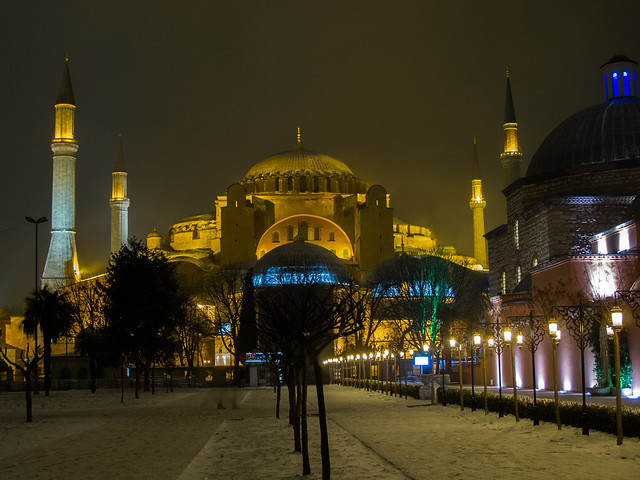This nighttime outdoor photograph captures a striking cityscape featuring a large, centralized building that appears to be a mosque, displaying Middle Eastern architectural elements. The main structure is defined by a sizable dome on top, colored in brown and gray, with a pointed pole rising from its apex. Surrounding the dome are four tall, slender prayer towers—two on the left illuminated in blue, and two on the right glowing in yellow or orange, due to the lighting. The building and dome are predominantly gray, contrasting with the vibrant tower lights.

The image is taken from a street-level perspective, looking directly down a street lined with trees, street lamps, and additional urban structures, some with illuminated windows. Snow blankets the ground, adding a serene touch to the scene. Although the street is textured with patches of sand and brick walkways, it appears deserted, intensifying the sense of stillness. The setting's various light sources cast a warm, inviting glow, subtly highlighting elements of the architecture and tree foliage. Despite the somber ambiance, the majestic mosque stands as a radiant focal point against the night sky.